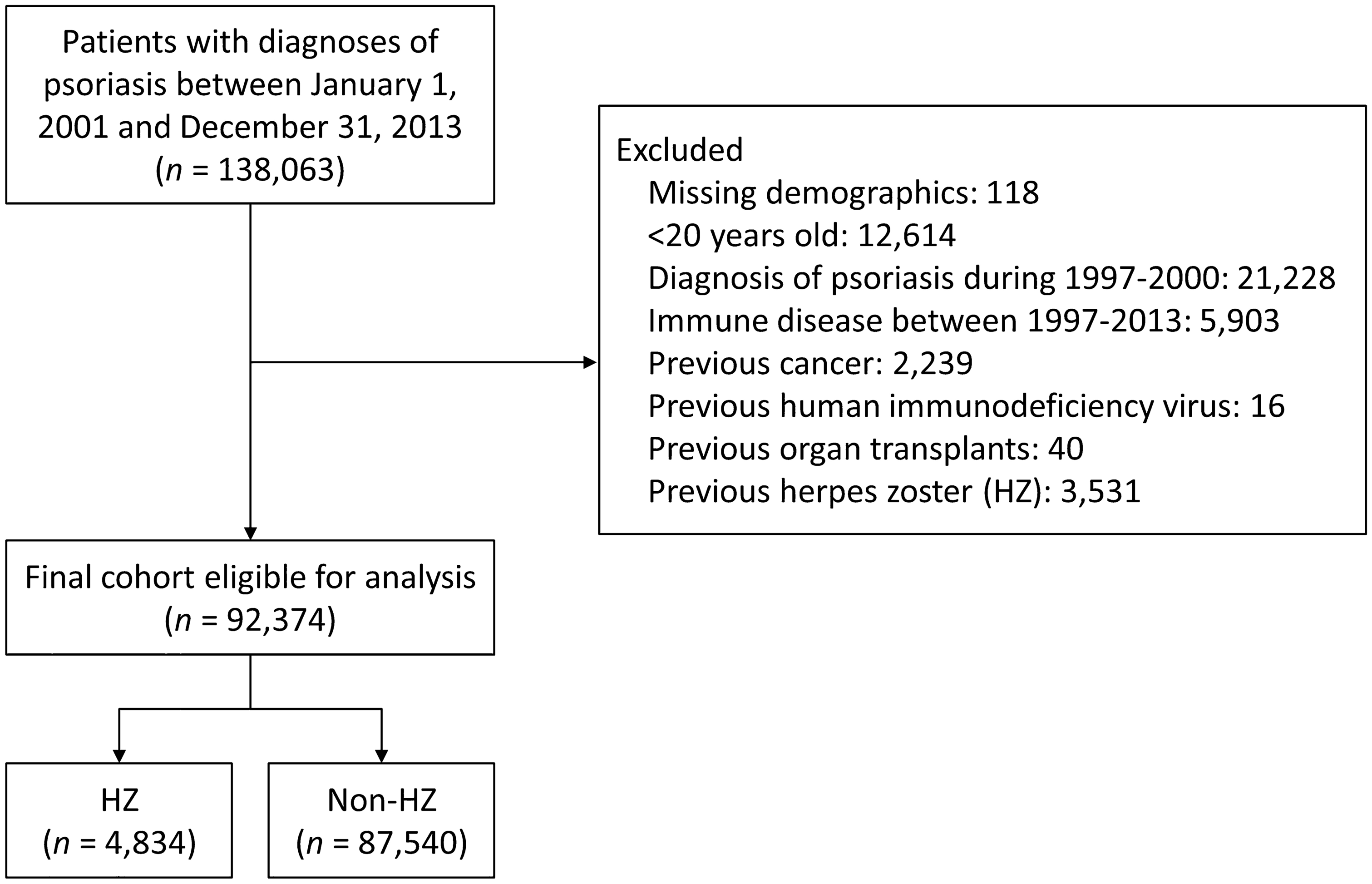The black and white image depicts a detailed flowchart from a medical study, primarily focusing on patients diagnosed with psoriasis between January 1st, 2001 and December 31st, 2013 (N = 138,063). The chart uses rectangular boxes connected by arrows to illustrate the process and grouping of data. The first box in the upper left corner states the initial patient group. An arrow from this box leads down to another box labeled "final cohort eligible for analysis" (N = 92,374). This box branches into two arrows pointing to separate boxes labeled "HZ" (N = 4,834) and "non-HZ" (N = 87,540). Additionally, from the first box, another arrow extends horizontally to a larger box marked "excluded," which lists criteria for exclusion such as missing demographics (118), age below 20 years (12,614), diagnosis of psoriasis between 1997-2000 (21,228), immune diseases between 1997-2013 (5,903), previous cancers (2,239), previous HIV (16), previous organ transplants (40), and previous herpes zoster (HZ) (3,531). The flowchart is visually coded in black and white text boxes, typical for medical or scientific documentation.